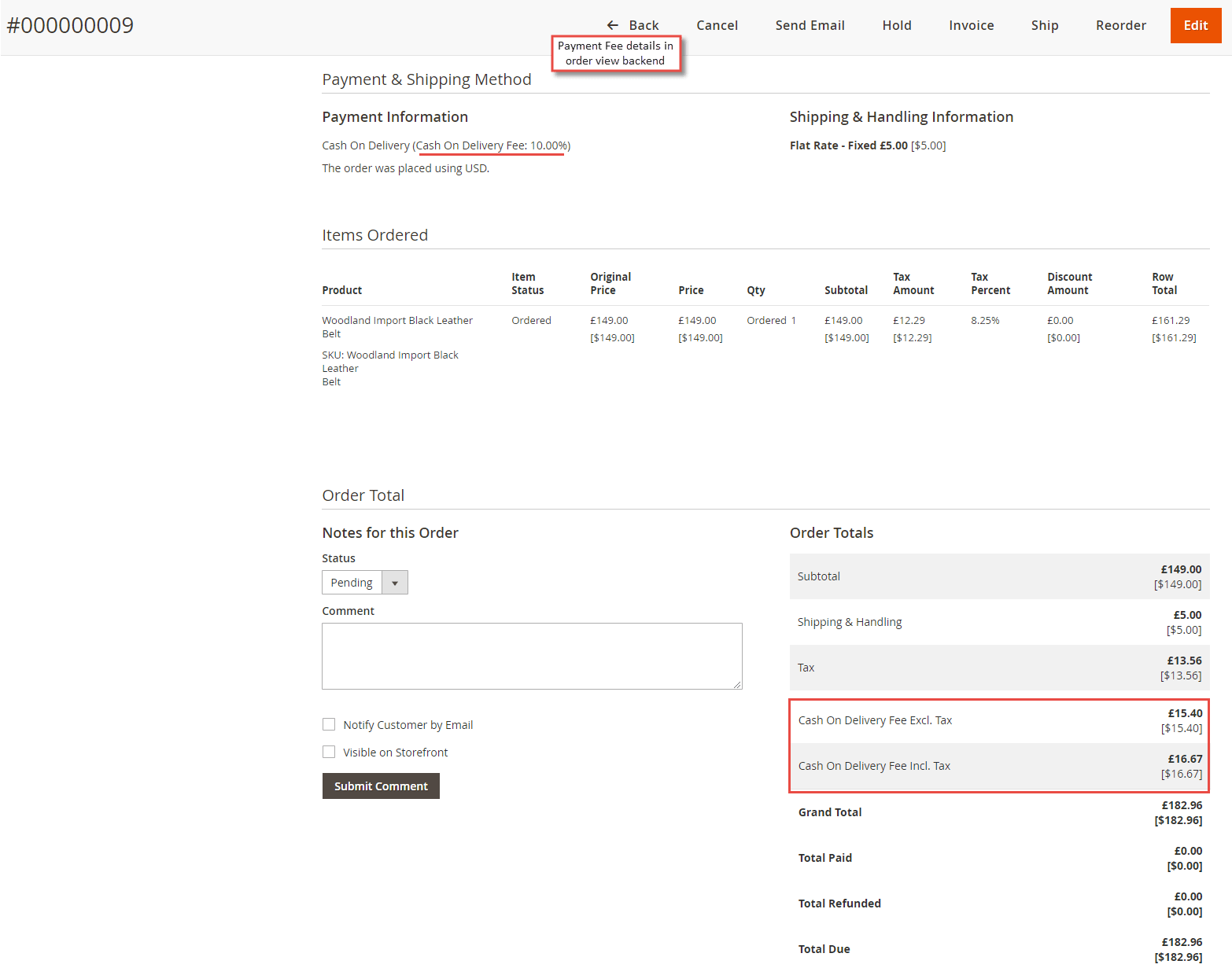**Descriptive Caption for Web Page Image:**

The image shows a detailed web page interface for managing payment and shipping methods on a website. The top banner is light gray, prominently displaying a number with a pound symbol: `0000009`. To the right of the number, there are several functional buttons including back arrow, tab, cancel, send email, hold, invoice, ship, record, and an orange edit button.

Underneath the banner, the section is split into two primary columns. On the left, the "Payment Information" section specifies the accepted payment method as "Cash on Delivery" with a fee noted at "10%". Also included is a timestamp whose specifics aren't legible.

On the right column, the "Shipping and Handling Information" is detailed, listing methods such as "Flat Rate" with fixed costs of 5 euros and 5 US dollars.

Below these sections, there is a structured table labeled "Items Ordered" which spans horizontally, segmented into categories from left to right: product, item status, original price, price, quantity, subtotal, tax amount, tax percent, discount amount, and row total. Product listings underneath this header include woodland import deck and leather items, though some details are illegible.

Following the items is a summarized "Order Total" section, and beneath it, a field for "Notes for This Order" featuring a drop-down menu for status options like 'pending', a comment input box, and checkboxes for notifying the customer by email and making the note visible on the storefront. The section concludes with a black "Submit Comment" button.

On the far right, an "Order Totals" summary panel is displayed. It includes subtotals for "Subtotal," "Shipping and Handling," and "Tax." Further highlighted in a red-bordered box are details for the cash on delivery fee both excluding and including tax. The final figures presented are the "Grand Total," "Total Paid," "Total Refunded," and "Total Due."